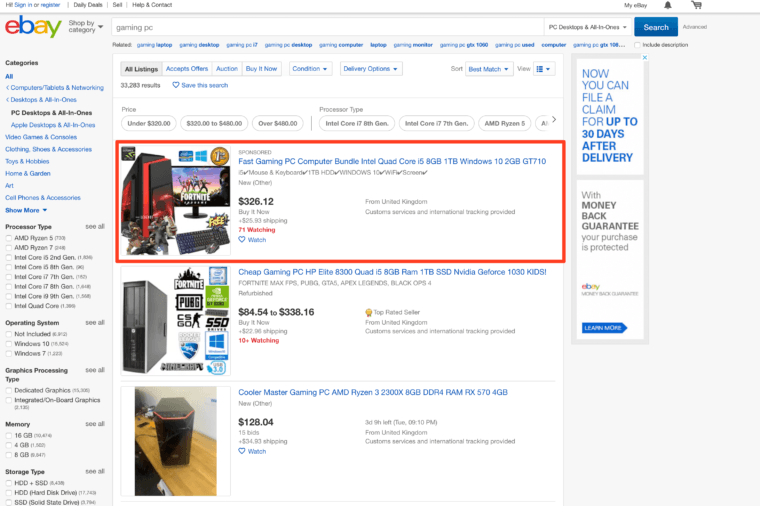Screenshot of an eBay search results page for "gaming PC" displayed on a computer. Highlighted in a red rectangle is the top listing, showcasing a red and black gaming PC tower, accompanied by a monitor, keyboard, and mouse. The description reads: "Fast Gaming PC Computer Bundle with Intel Quad-Core i5, 8GB RAM, 1TB HDD, Windows 10, 2GB GT 710," priced at $326.12. On the left is a grey sidebar with category filters, where "PC Desktops & All-In-Ones" is the only selected option. Two additional search results are visible below the highlighted listing.